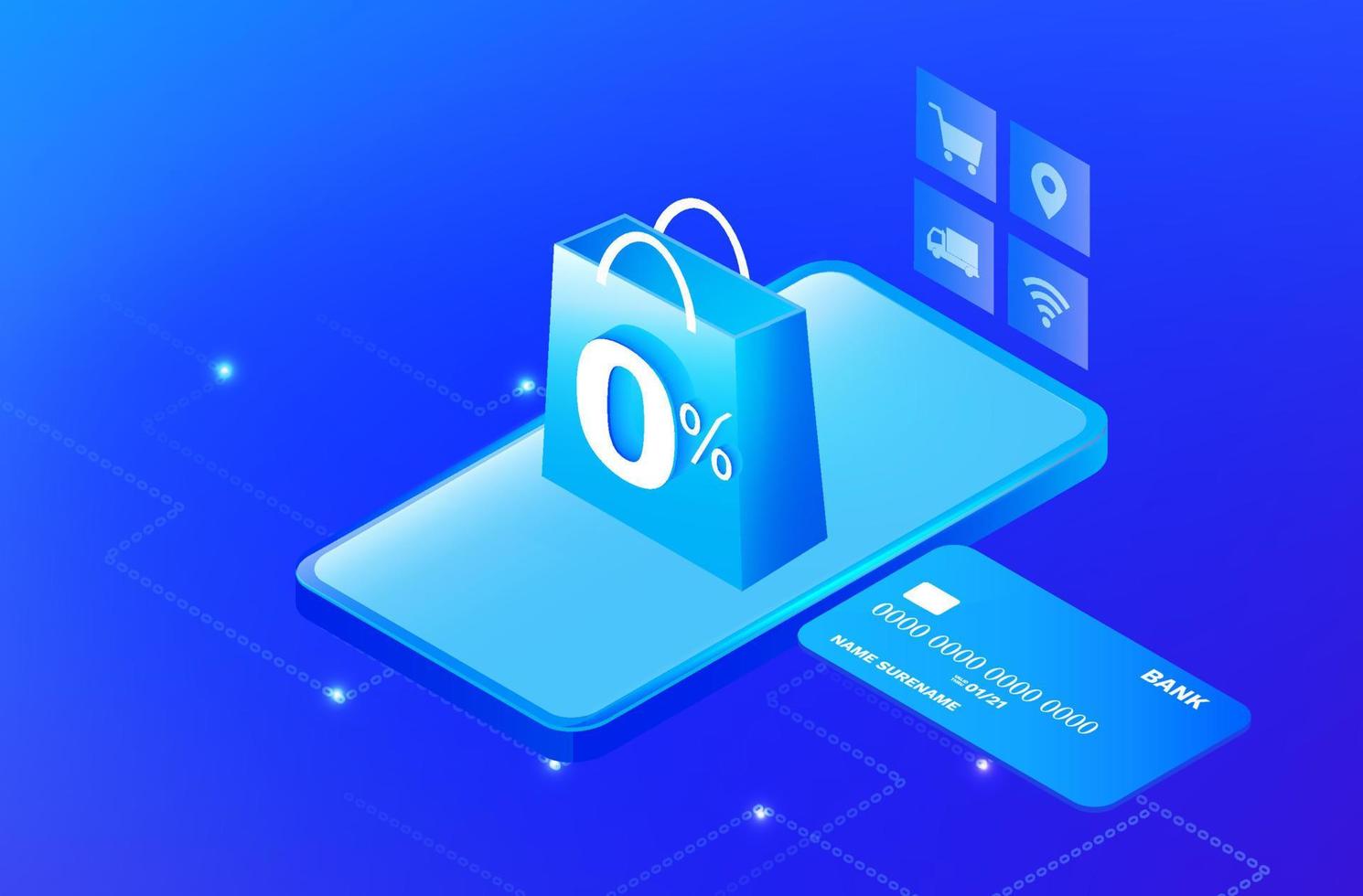The digital graphic features a smartphone at the center, prominently displaying a 0%-marked shopping bag on its screen. To the right of the smartphone is a generic, unbranded bank card with placeholder numbers and names, signifying a typical demonstration card. Above the smartphone screen are four key icons: a shopping cart, a location pin, a delivery truck, and a WiFi signal. The image employs a monochromatic color scheme dominated by purple and blue tones and has a clean, computer-generated style typical of stock images used across various apps, websites, and news articles. The flat blue background and blue platform further emphasize the promotional nature of the image, likely intended for a financial institution or a credit card company. The visual elements suggest a streamlined online shopping experience, guiding users through the process of adding items to their cart, choosing delivery options, and entering payment details.